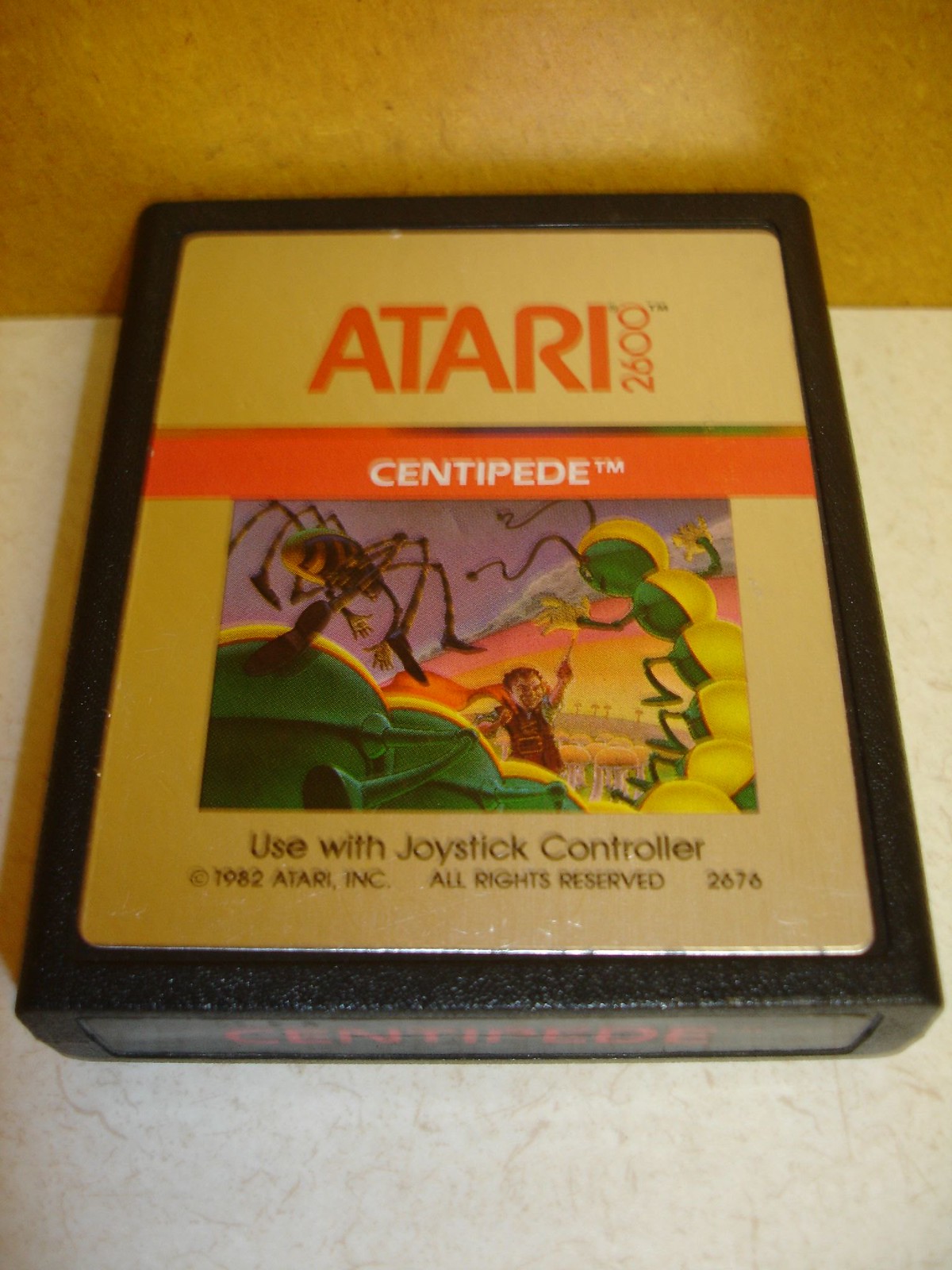This photograph captures an Atari 2600 game cartridge resting on a linoleum surface. At the top edge of the image, the linoleum displays an orange stripe, while the lower part features a mix of gray and beige tones, though the exact colors are difficult to discern due to poor lighting. The central focus of the image is the black Atari cartridge, adorned with a silver label. Prominently written in red on the label is "Atari 2600." Below this, a red bar with white text reads "Centipede™". The cartridge artwork depicts a dramatic scene where a giant green and yellow centipede menaces a tiny elf-like man, who bravely brandishes a gun while standing on a hill. A caption below the graphic states "Use with joystick controller" in black font.